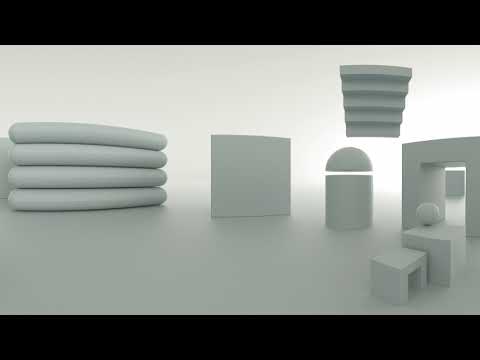The image depicts an all-white, minimalistic room with various shapes and symmetrical objects arranged throughout. The room is brightly lit, accentuating the monochromatic color theme of white and light gray. On the left side, there are four stacked rectangular pillows or towels, followed by a medium-sized square shape. Adjacent to this, there is a small cylindrical object topped with a dome-like half-circle. Suspended in mid-air above these objects is an upside-down staircase leading to nowhere. To the right of these items, there is a square-shaped doorway, through which another square shape is visible. In front of this doorway, a white square box sits with a sphere resting on top of it, accompanied by another small square shape. The entire composition features an array of shapes and sizes, creating an intriguing yet simple visual narrative dominated by white hues.